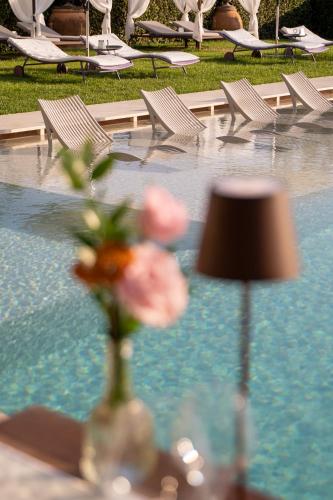The image captures an inviting outdoor scene centered around a serene swimming pool. In the foreground, a small, blurred lawn area adorned with vibrant pink and orange carnations mixed with lush greenery can be seen, accompanied by a miniature lamp likely designed to house a tea light. The pool itself boasts a calming blue hue and features a sun shelf with four reclining chairs slightly off in the distance. Surrounding the pool, a glass barrier runs the length of the decking area, contributing to the modern aesthetic. Behind the glass, several adjustable loungers with wheels on their backs are arranged for optimal relaxation. Additionally, there is a hint of a cabana, indicated by pieces of cloth attached to its corners. The photo, taken during the daytime, showcases clear reflections on the tranquil water's surface, enhancing the overall peaceful ambiance. Notably, the image contains no text or writing.